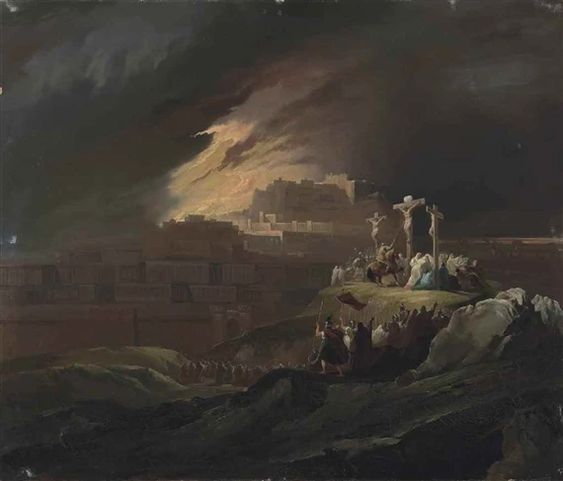The painting captures a dramatic and somber scene of three crucifixions set against a turbulent, dark gray sky that hints at an impending storm. The center figure, likely Jesus, and two others are affixed to crosses by their hands and feet, wearing only loincloths. Dominating the foreground is a hill with numerous onlookers, including a man on horseback holding a spear poised to pierce the side of the figure on the central cross. Surrounding this central action, several soldiers clad in red cloaks brandish red flags, some standing, others kneeling, their expressions and body language conveying a range of emotions from shock to reverence. Behind this poignant tableau, a multi-tiered cityscape with flat-roofed stone buildings and the imposing walls of Jerusalem stretches into the background. The overall composition is painted in dark, moody tones, enhancing the painting’s ancient and solemn atmosphere.